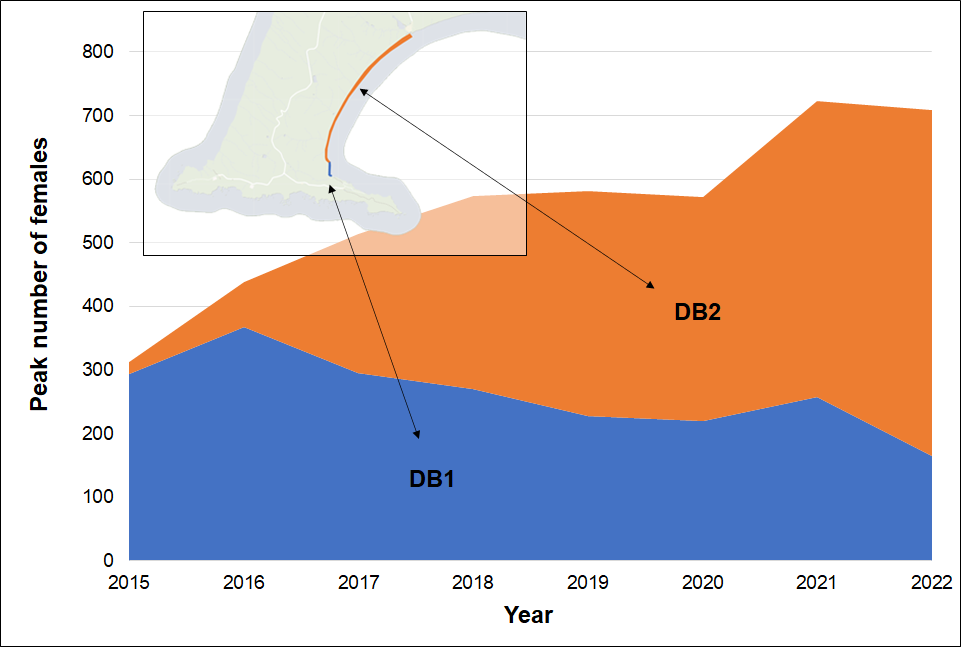This image features a detailed graph with a black border, illustrating the peak number of females over a span of years from 2015 to 2022. The vertical axis on the left ranges from 0 to 800, incremented by hundreds, and represents the peak number of females. The horizontal axis at the bottom designates the years from 2015 to 2022. The graph includes two distinct data sets: DB1, depicted in blue, and DB2, shown in orange. DB1 data points lie at the bottom part of the chart, while DB2 data points are positioned in the upper section. Additionally, there is a highlighted box indicating a notable rise in the data, with an arrow pointing to a segment of the blue DB1 dataset, showcasing its relation to the orange DB2 data. The graph is set against a white background, emphasizing the distinctive colors and layout of the data.